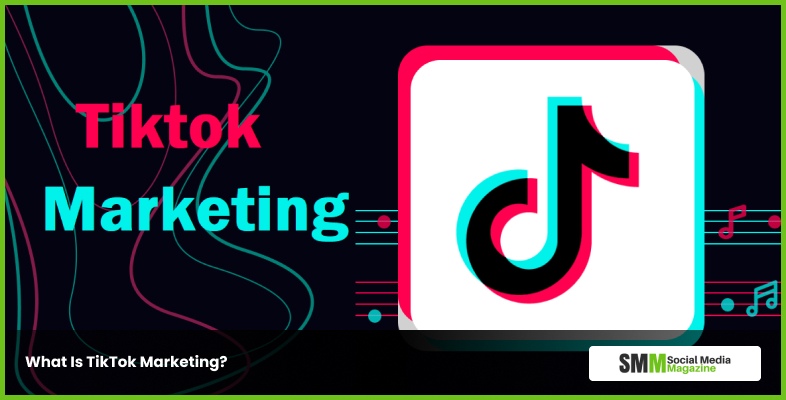A colorful and visually engaging webpage prominently features a landscape-oriented image on a white background. On the left side, "TikTok" is written in red at the top, followed by "Marketing" in a vibrant aqua blue underneath. The background of this section is adorned with dynamic, wavy lines that mainly move vertically, with one notable blue line that curves from the top, swoops down about one-third of the way, and then ascends again.

At the bottom left corner, the question "What is TikTok Marketing?" is displayed. The right side of the image showcases the iconic TikTok logo—a stylized music note in black, blue, and red. This logo stands out against a background that transitions from reddish hues at the top and left to light blue hues at the bottom and right. Centered behind the TikTok logo is a music score with alternating blue lines and red notes, which inversely transitions to red lines with blue notes near the bottom.

Below this musical motif, a white background section contains the text "SM" in black followed by "M" in green. The labels "social media" and "magazine" are written below in a smaller font size, with "social media" in black and "magazine" in green, respectively. This detailed and structured design effectively captures the essence of TikTok marketing within a visually appealing layout.